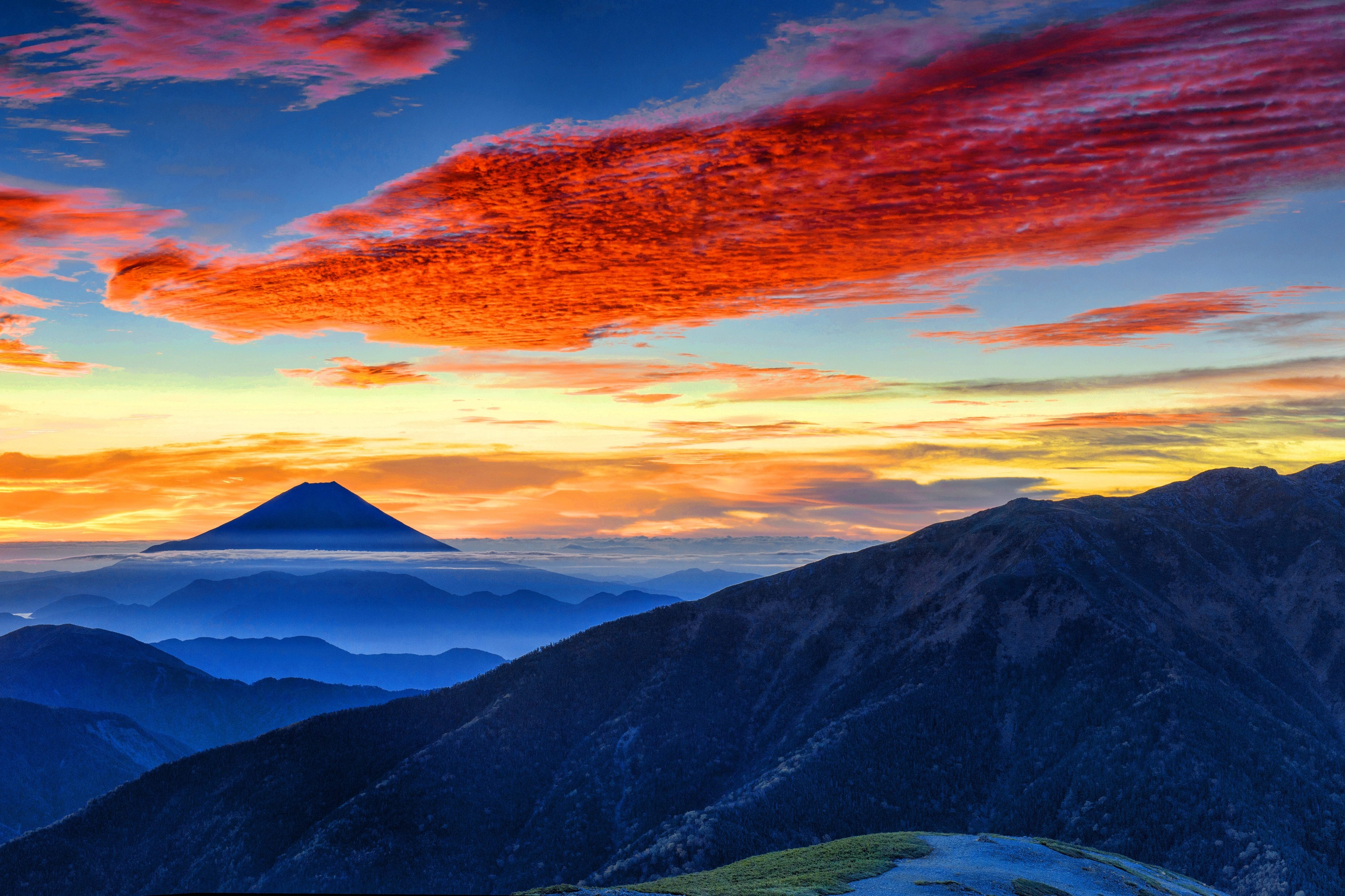The image captures a mesmerizing mountainous landscape that could be a photograph or an exquisite painting. Dominating the background, a large blue mountain or possibly an ancient temple rises up, enveloped in a blue mist that accentuates its enigmatic presence. The view is taken from a high vantage point on a rocky mountain, framed by a series of jagged mountain ridges that stretch into the distance. The sky is a spectacular blend of colors, suggesting either dawn or dusk, with clouds vividly lit from below. These multicolored clouds transition from a warm yellow near the horizon to a rustic, light blue and finally to a rich red as they approach overhead. The foreground features a rocky outcropping and scattered patches of green grass, contrasting beautifully with the cooler, bluish hues of the distant ridges and the possible snow caps on the higher peaks. The entire scene evokes a serene and awe-inspiring atmosphere, free from the presence of people or any inscriptions.